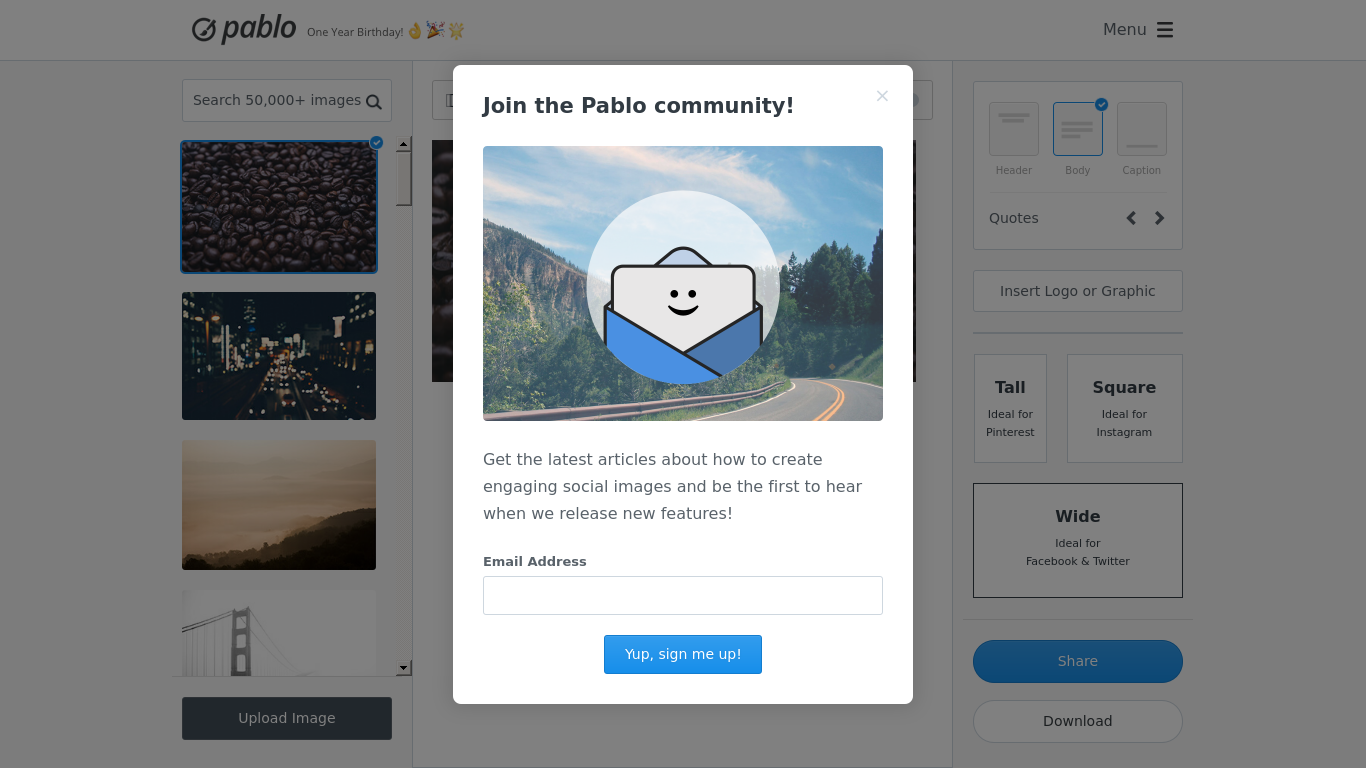**Detailed Caption:**

The screenshot captures a pop-up window designed to encourage users to join the Pablo community. Positioned at the top, the header reads "Join the Pablo Community," emphasizing the call to action. Above this text is a serene image featuring a long, winding road traversing through mountainous terrain, creating an inviting and adventurous ambiance.

Superimposed on the scenic picture is a circular icon resembling a letter envelope adorned with a friendly smiley face, adding a touch of warmth and approachability to the visual. Below the invitation text, the pop-up clearly states: "Get the latest articles about how to create engaging social images and be the first to hear when we release new features," appealing to users who want to stay updated on valuable tips and product enhancements.

Further down, there's a prompt asking for the user's email address, accompanied by an empty text box where the email can be entered. Following this input field, a prominent blue button labeled "Yep, sign me up" invites users to complete the subscription process.

In the backdrop, the remainder of the webpage is subtly visible, hinting at a site filled with high-quality stock images, which aligns with the context of creating engaging social images.